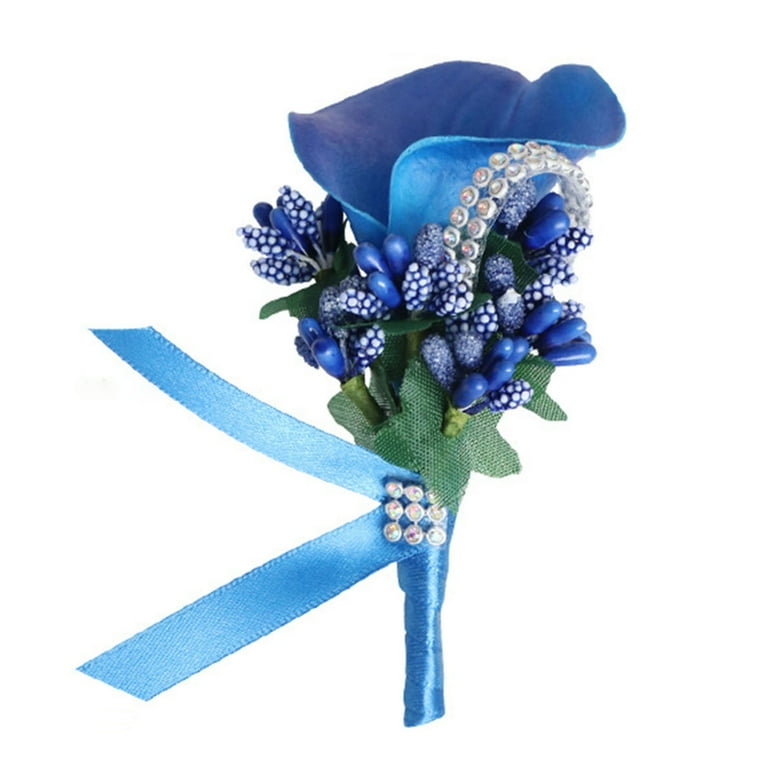This vibrant and intricately detailed image showcases a handmade blue corsage, perfect for a formal event. At the top of the corsage is a striking, large blue lily flower made of satin material. Beneath it, a cluster of blue beads and decorative foam bulbs, some solid blue and others with blue and white polka dot patterns, resemble seeds or capsules. Adding a touch of sparkle, a bracelet-like string of craft rhinestones peeks out from under the petals. Surrounding the flower, there is a mesh made from green gauze that mimics the appearance of leaves, adding to the floral impression.

The stem of the corsage is wrapped in a light blue ribbon that culminates in a bow, which is further adorned with a cluster of nine rhinestones, enhancing its decorative appeal. The overall theme features hues of light blue and royal blue, creating an elegant and cohesive look.